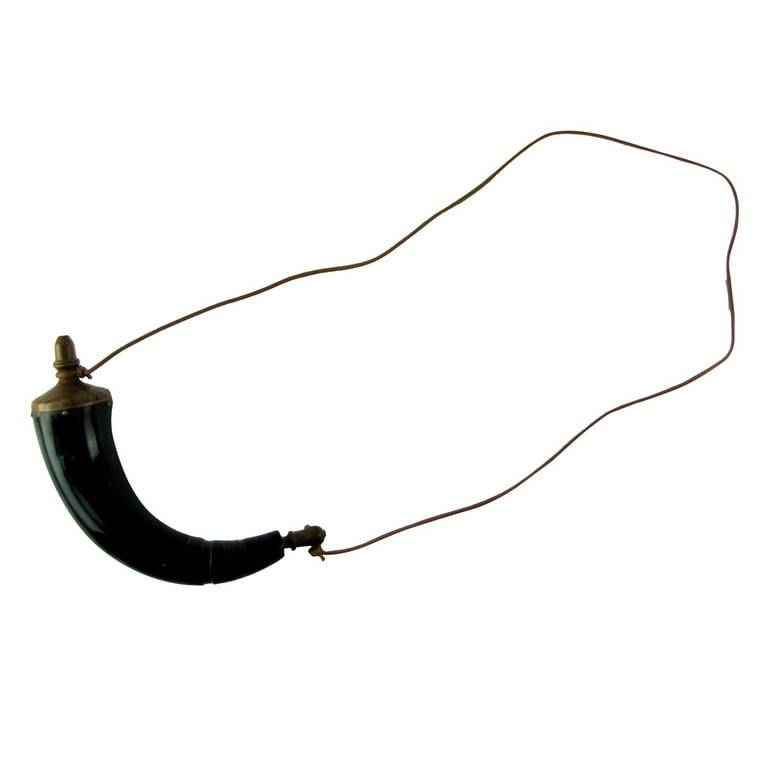The image depicts a detailed photograph of an amulet-like vessel, reminiscent of a polished, jet-black animal horn or curved metal piece. Measuring approximately two inches in length, the horn-shaped item is adorned with brass or coppery accents forming small caps or knobs at both ends. A sturdy black string is securely tied around these knobs, allowing the vessel to be worn around the neck. The dark, shiny surface of the vessel suggests it has been painted or finished to enhance its appearance. One end appears to have a small, twist-off cap connected to the string, possibly indicating its function as a container, perhaps traditionally used to hold liquids. The object is presented against a stark white background, highlighting its intricate and polished details.